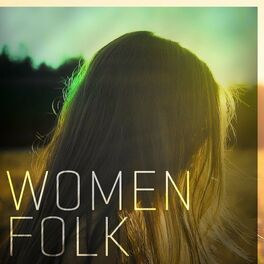The image features a square photograph, likely an album or CD cover, showcasing a woman with long, possibly blonde or brown hair, cascading down and obscuring her face. She is oriented to the right side of the image, with her right shoulder partially visible. In the background, a landscape of dried grass stretches out, dotted with green trees. The sky above carries a grayish-green hue, and sunlight appears to be shining down on the woman. In the bottom left corner, the title "WOMEN FOLK" is displayed in a thin, white, all-caps font, with "WOMEN" on the first line and "FOLK" directly beneath it.